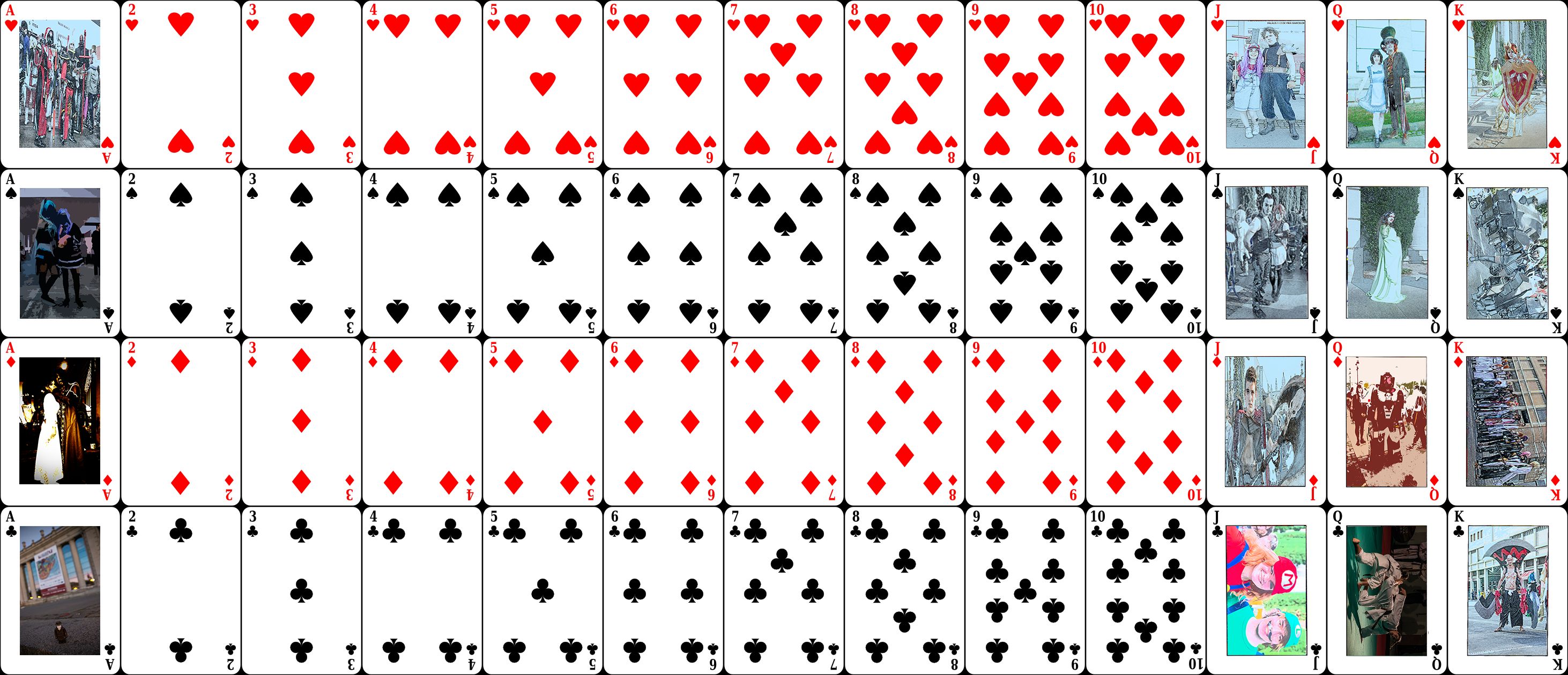The image displays a meticulously arranged collection of playing cards, organized by suit in four horizontal rows. The top row features the hearts suit, presented in sequential order from Ace to King. Each card reveals both its face and back design. The subsequent row showcases the spades suit, similarly arranged from Ace to King. The face cards—Jack, Queen, and King—are adorned with intricate illustrations, as is the Ace of Spades, albeit the details are minute.

The third row consists of the diamonds suit, arrayed from Ace to King. Following this, the bottom row exhibits the clubs suit, also organized from Ace to King. Each suit's face cards—hearts, spades, diamonds, and clubs—distinctly feature individual illustrations for the Jack, Queen, and King. The image provides a comprehensive and detailed view of the entire deck, highlighting both the uniformity and the unique artistic elements of the face cards in each suit.